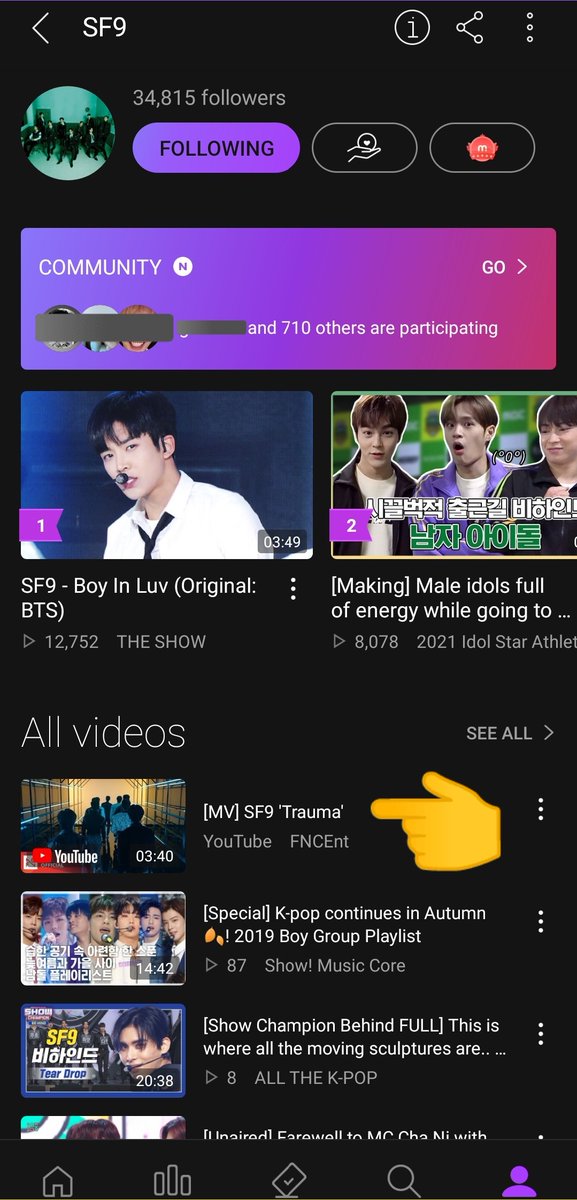This is a detailed screenshot taken from a mobile website. The screen has a black background with a white greater-than sign pointing to the left located at the top left corner. To its right are the characters "SF9" in uppercase. On the right side of the screen, there are three vertically aligned white circles, followed by a red, yellow, and white share button. Below these, there's a black circle with a white border enclosing a white number "1".

On the left side of the screen, there's a circular profile picture featuring a gray background and four or five men dressed in black. To the right of the profile picture, it indicates "34,815 followers." Directly underneath this is a purple tab labeled "Following" in black text. Adjacent to it, there is a black tab with a white border displaying an icon of a hand holding a heart, followed by another black tab with a white border encompassing a red circle with a white "M" on it.

Beneath these elements, a horizontally aligned rectangle transitions from purple on the left to pink on the right with the word "Community" written in white, next to a white circle with a black "N" inside. The right side of this rectangle has a white "Go" label.

Continuing downward, there is a section indicating that profile pictures are blocked out. At the middle of the screen in white text, it states, "...and 710 others are participating." Below this, there are two images side by side labeled as videos. Information about these videos is provided underneath.

Further down, the screen displays "All Videos" on the left and "See All" in smaller letters on the right. Below this section, three profile pictures are aligned horizontally, correlating with videos. To the right is additional information about these videos. The first profile picture on the right includes a prominent emoji hand pointing to the left.